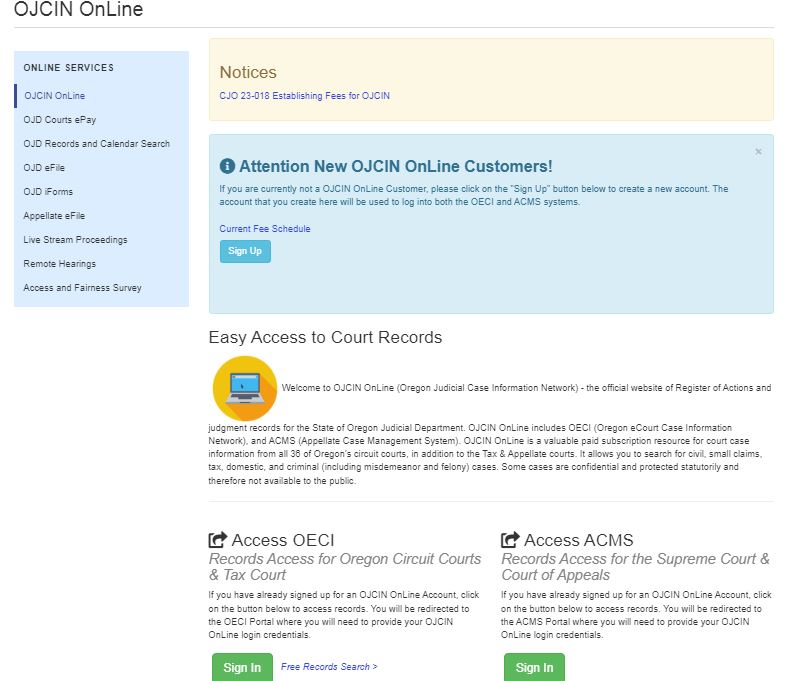The website displayed is OJCINonline, featuring a clean layout with black font on a white background. A prominent blue rectangle, taller than it is wide, is centrally located and lists various online services in white text. These services include: Online Services, OJCINonline (highlighted), OJD Court ePay, OJD Records and Calendar Search, OJD eFiles, OJD iForms, Appellate eFile, Livestream Proceedings, Remote Hearings, and Access and Fairness Survey. At the top, a notice in bold text states, "CJO23-018 Establishing Fees for OJCIN." It also addresses new users with a message: "Attention new OJCINonline customers. If you currently are not an OJCINonline customer, please click on the Sign Up button below to create a new account." This account will be used for logging into both the OECI and ACMS systems. The message is set against a blue background.